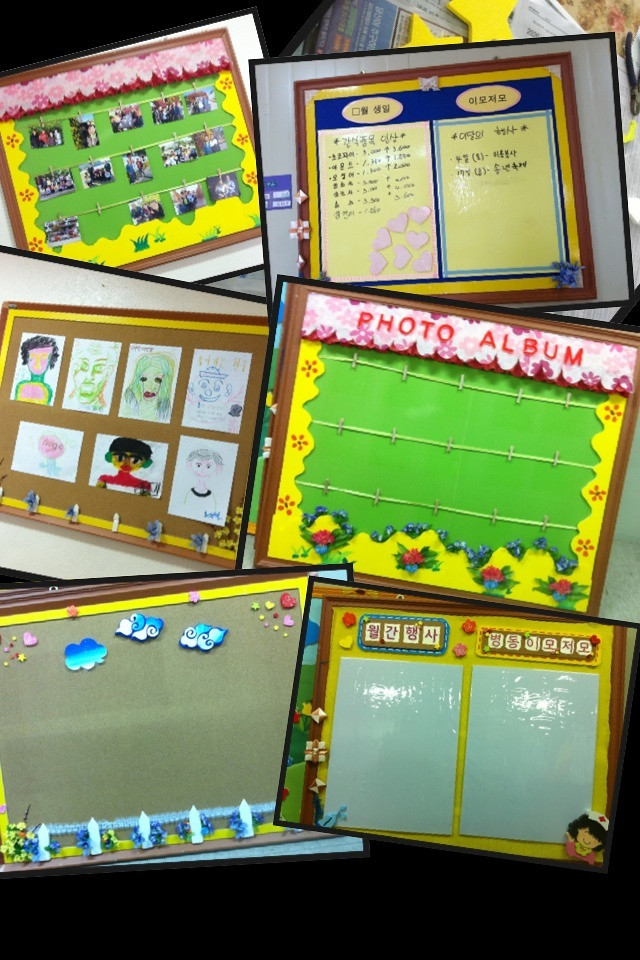The photograph depicts a vibrant and eclectic display of six bulletin boards, characteristic of an early grade school or kindergarten classroom. The boards are arranged at various angles, creating a dynamic and engaging collage. Each bulletin board features distinct themes, styles, and colors ranging from pink to green and yellow.

The top left bulletin board showcases small photographs hanging from three yellow lines against a backdrop adorned with red and green shapes. Next to it is a bilingual menu-like display with a blue top and yellow bottom, separated by blue borders into two lists; the text appears in an Asian language. Another board highlights children's artwork with a mix of green, red, and blue hues, evidencing youthful creativity. 

On the bottom right, a board features what appears to be magic drawing slates accompanied by Asian-style scrabble cubes and a depiction of a school nurse, centered within shiny rectangular white areas. Adjacent is another colorful display, which includes a sports field illustrated with strings and staples, bordered in yellow. Additionally, there is a gray-background board to the left with three clouds, likely used for weather-related educational purposes.

Overall, the intricate assembly of these bulletin boards, with elements such as the "Photo Album" heading on a pink background and various children's drawings, captures the lively essence of a classroom environment.